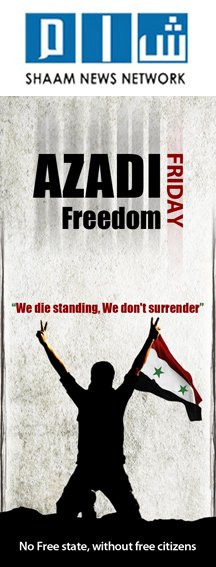This is a vertical, color image that appears to be an advert for a TV channel called Sha'am News Network, spelled S-H-A-A-M. At the top of the image, there are three blue boxes, each containing a white symbol. Below that, the words "Sha'am News Network" are written in black font. Dominating the center of the image, there is a silhouette of a man on his knees with both arms raised. He is holding a flag that is red, white, and black with green stars, possibly the Palestinian flag. Above the silhouette, the text reads "Azadi Freedom Friday" (A-Z-A-D-I). In the middle of the image, a quotation states, "We die standing, we don't surrender." At the very bottom, beneath the silhouette, it says in white font against a black background, "No free state without free citizens."